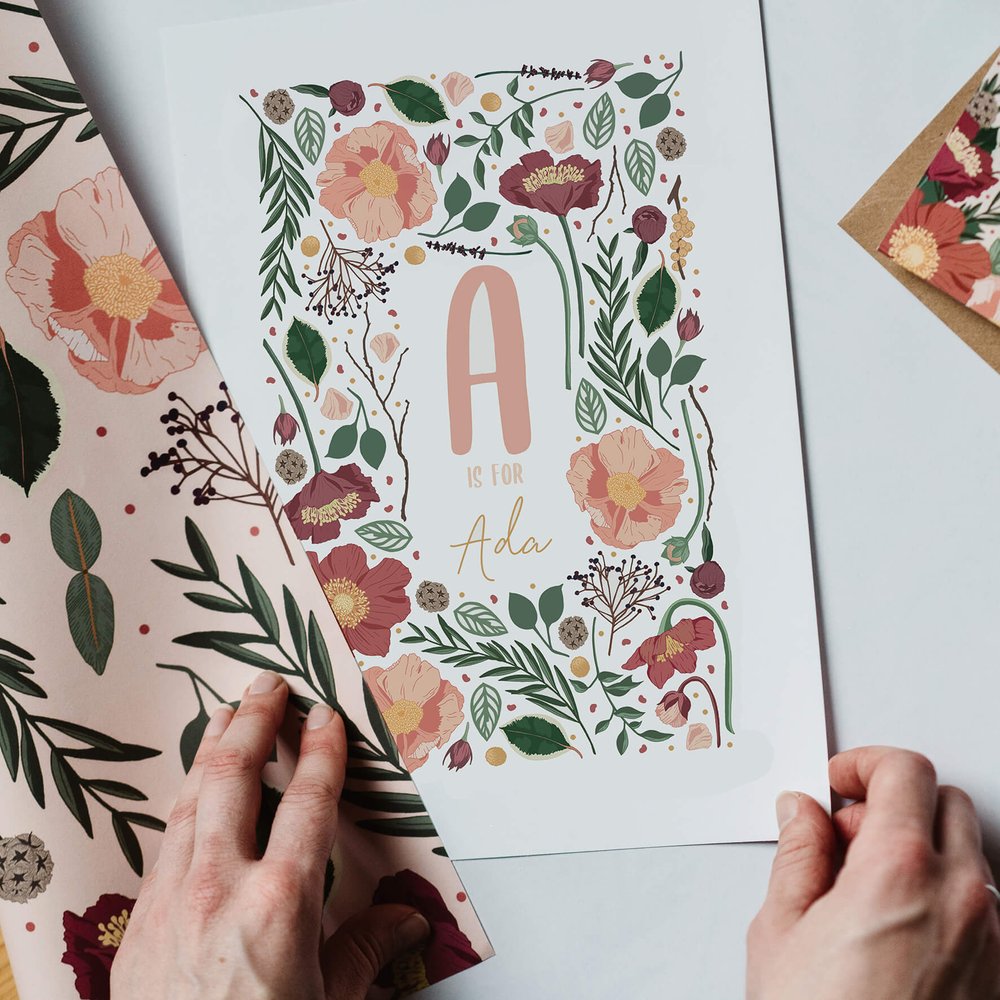The image captures a person placing a carefully designed scrapbook page, with their hands visible at the bottom right and bottom left of the frame. Central to the scene is a white paper adorned with an assortment of pink flowers with green leaves and stems, arranged in a variety of styles. Dominating the center of the page is a bold, pink letter "A," beneath which, in smaller capital letters, it reads "IS FOR," followed by "ADA" in delicate cursive. On the left side, part of another scrapbook page peeks into view, while the top right reveals the corner of a similar piece. Beneath these layers, a piece of textured, cardboard-colored paper slightly extends past the scrapbook pages, adding depth to the composition. The background appears to be a plain white surface, emphasizing the vibrant floral designs and intricate lettering.